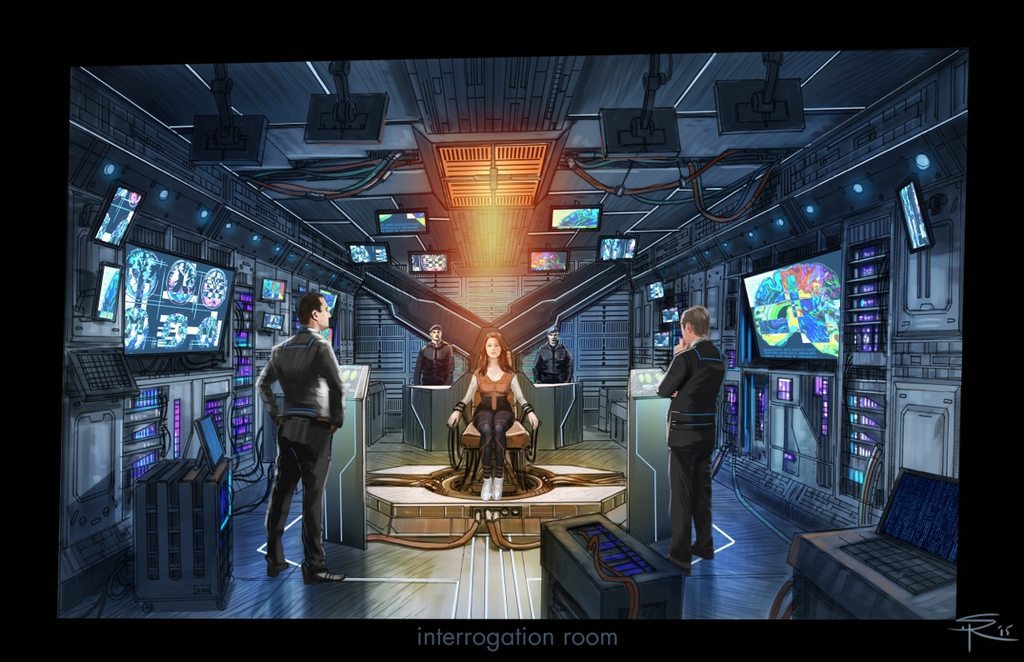In a futuristic, cartoon-styled image, a woman is seated in a central chair under a red light, signifying its importance. She appears restrained, her arms tied down, as she is being intensely examined by four men in suits and uniforms, who surround her from four different angles. The room is filled with numerous screens, including at least four in the foreground and more in the background, displaying bright images, potentially of her brain. The scene is richly detailed, resembling the interior of a spaceship, with multiple pillars and a unique floor. Above, at the bottom of the scene, "Interrogation Room" is written in white on a black strip, with "R 12" noted beneath it.